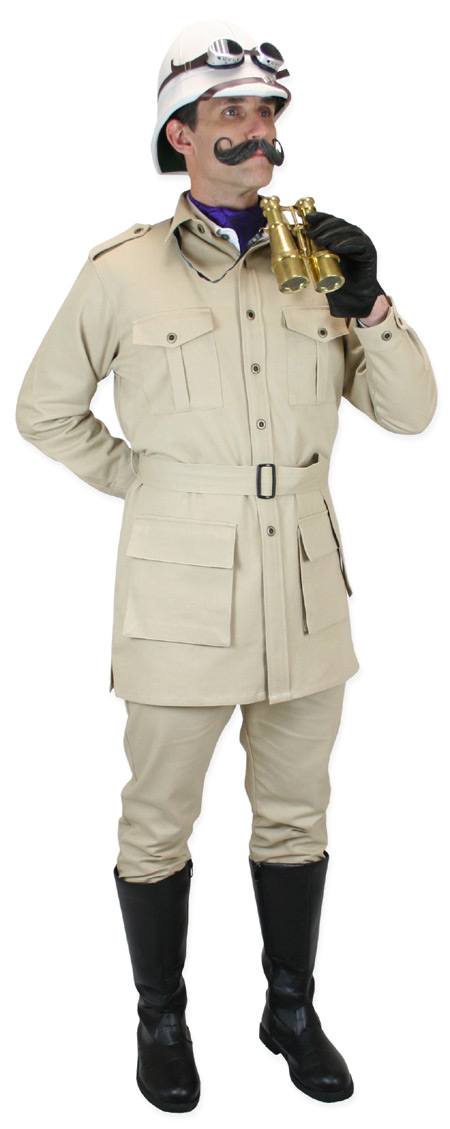The image depicts a vertically-oriented, highly stylized photograph of a Caucasian man standing centered in a pure white void, contributing to the notion that it is a stock photograph. The background is completely white, without any objects or text. The man is dressed in an outfit reminiscent of an early 1900s or late 1800s explorer or military dress uniform. 

He wears a distinctive tan coat, extending from his shoulders down past his hips to about mid-thigh, featuring black buttons down its length, a belt at the waist, and side pockets beneath the belt. Beneath the jacket, a touch of purple fabric is visible. He pairs the coat with matching tan pants, tucked into knee-high, heavy black rain boots. 

The man sports a prominent, curly handlebar mustache and wears a white helmet with a slight brim that curves around his forehead, down over his ears, and towards the back of his neck. A pair of goggles with a black strap rest atop the helmet. 

In his right hand, he holds a pair of golden binoculars around neck level, pointed downward, while his left hand is positioned behind his back, wearing a dark brown glove. His blue eyes gaze forward, enhancing the classical explorer or military aesthetic of the scene.